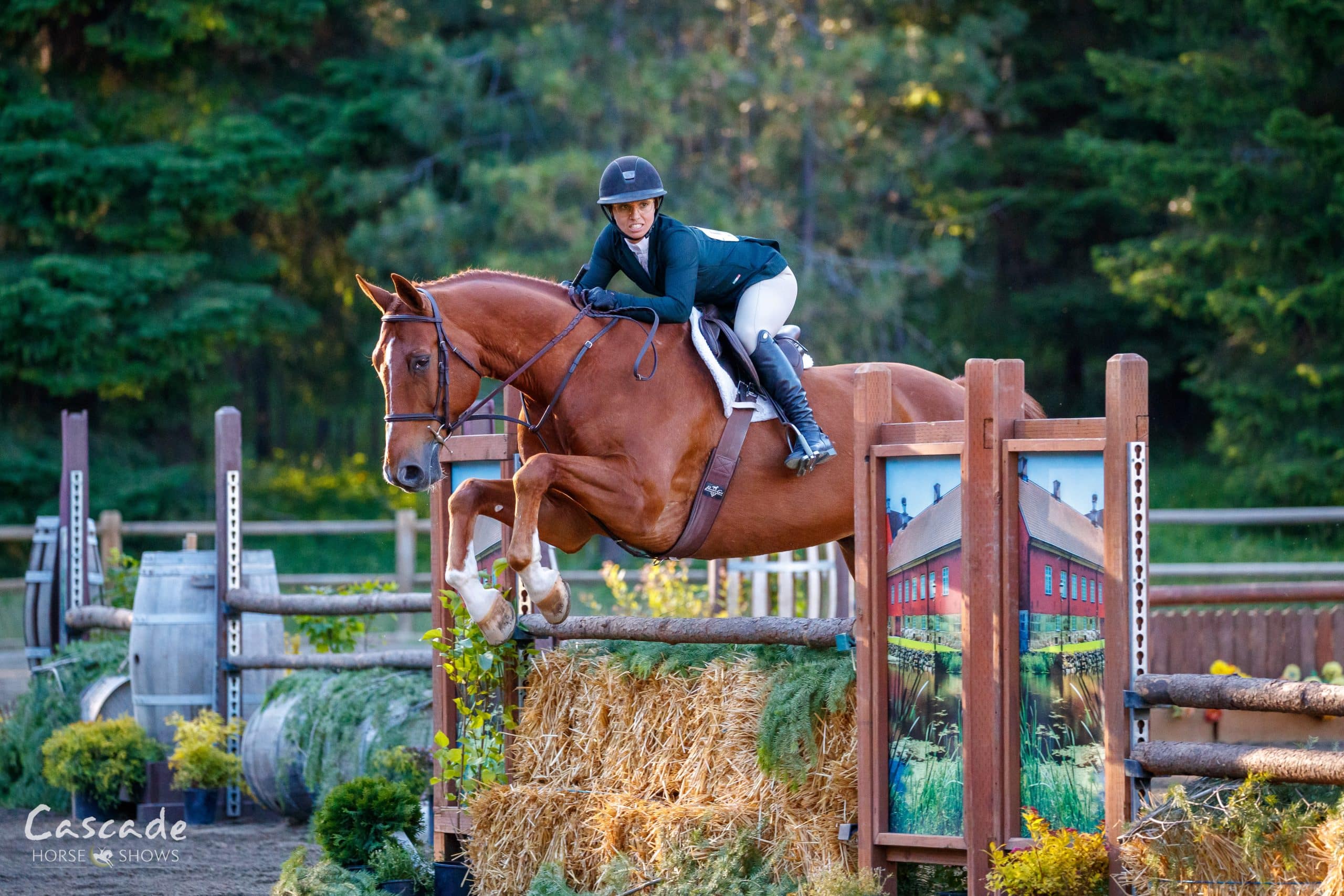In this dynamic and captivating photograph from Cascade Horse Shows, a chestnut-colored horse with a neatly groomed short mane and white stockings is captured mid-leap over a hurdle. The hurdle is uniquely constructed with a real tree branch supported by a hay bale and two fences, which are adorned with painted images of a red barn. The female jockey, equipped with a black helmet, a blue blazer, white trousers tucked into long black leather boots, and a white shirt, is perfectly poised on the horse's back, looking determinedly towards the camera. The scene resembles a steeplechase race, with various obstacles such as barrels and plants scattered along the racetrack. In the background, a thick forest with tall, out-of-focus trees frames the action, emphasizing the rider and the horse's leap. The bottom left corner of the image sports the stylized font reading "Cascade Horse Shows," adding a promotional touch to this thrilling equestrian moment.